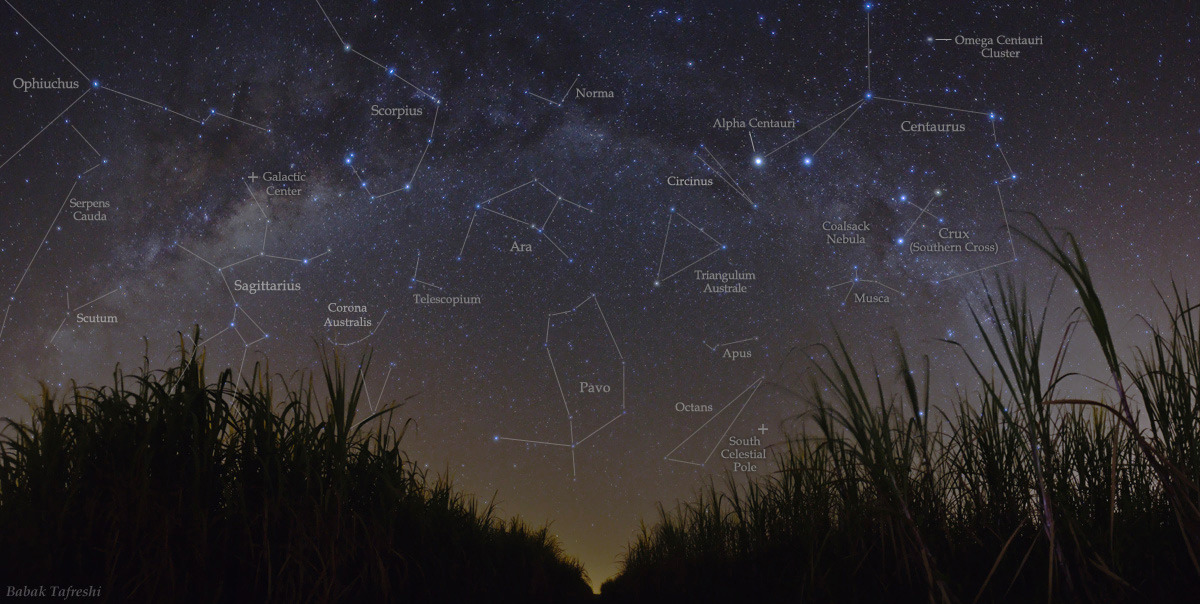In this nighttime image, the black sky is densely populated with twinkling stars, intricately showcasing identifiable constellations. Prominently, various stars are connected with fine lines forming distinct patterns, with some constellations labeled. Key constellations like Sagittarius, Ara, Pavo, and Musca, among others, are marked. The labels include Ophiuchus, Serpens Cauda, Scutum, Galactic Center, Corona Australis, Scorpius, Norma, Arrow, Telescopium, Alpha Centauri, Cercinus, Triangulum Australis, Apis, Octans, and the South Celestial Pole. The right side highlights Omega Centauri Cluster, Centaurus, Coalsack Nebula, Crux, Southern Crust, and Musca.

Beneath this celestial display, dark, grassy hills, detailed with tall grasses on the left and right, form the horizon. These hills gently slope across the foreground, merging with the star-filled expanse above. The scene is almost serene, with a faint hint of light illuminating the middle background, enhancing the night sky's mesmerizing appearance.